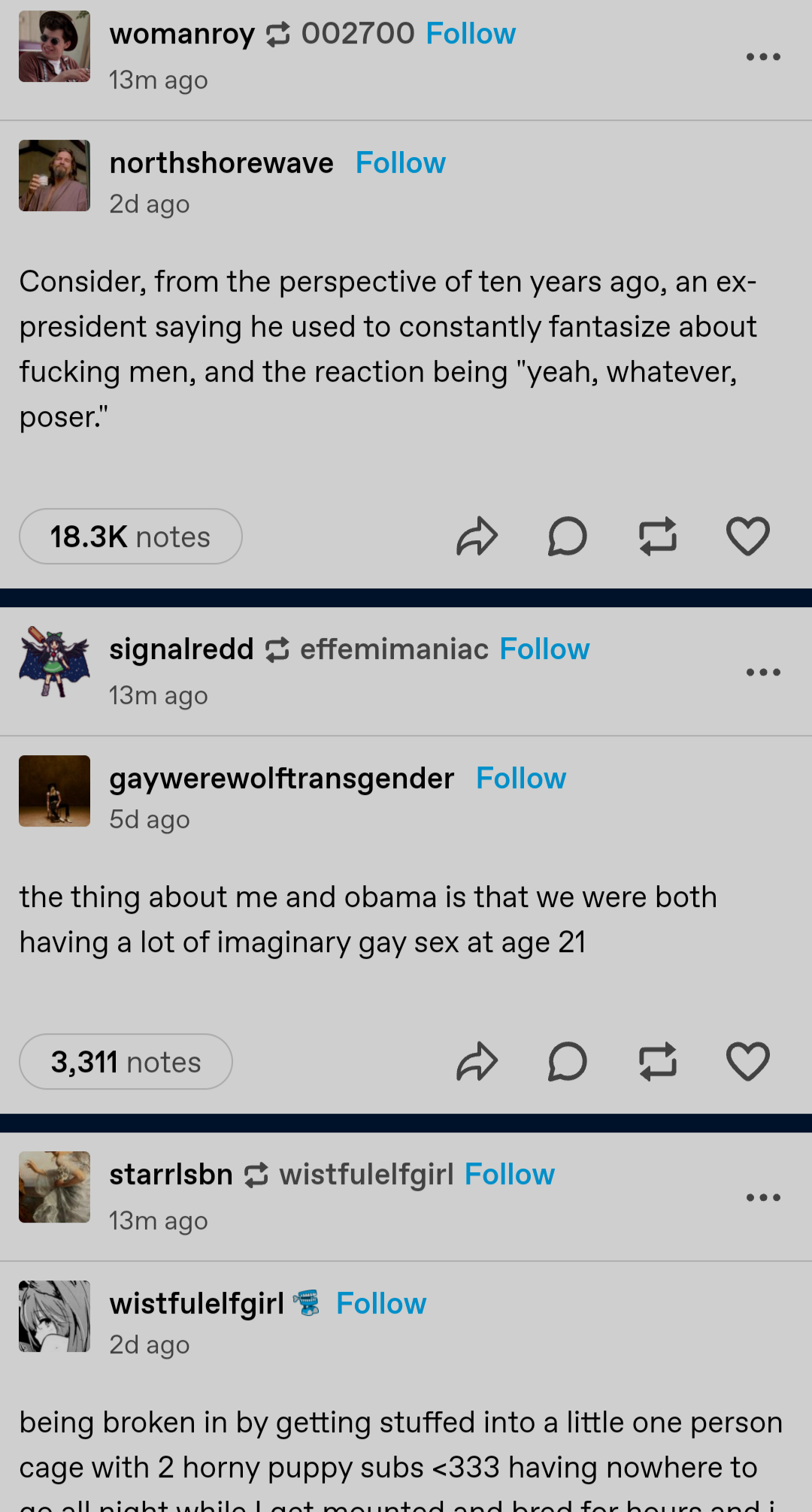Here's a cleaned-up and detailed caption:

---

The image captures a screenshot from a cell phone, depicting an activity feed with multiple posts. The background is a muted gray, with black lines delineating the sections. 

At the top of the screen, the user "Woman Roy 002700" is highlighted, featuring a blue "Follow" button next to the username. The text "13m ago" indicates the post was made 13 minutes ago.

The first post, labeled "North Shore Wave" from two days ago, reads: "Consider from the perspective of 10 years ago an ex-president saying he used to constantly fantasize about fucking men and the reaction being yeah, whatever poser." This post has garnered 18.3K notes.

Further down, a post by "Gay Werewolf Transgender" states: "The thing about me and Obama is that we were both having a lot of imaginary gay sex at 21," with 3,311 notes.

At the bottom, a partial post by "Wistful Elf Girl" appears with a follow button beside her username. The message reads: "Being broken in by getting stuffed into one a little one-person cage with two horny puppy subs Having nowhere to..." but cuts off before completing the thought.

---
This caption provides a thorough and structured description of the image contents.